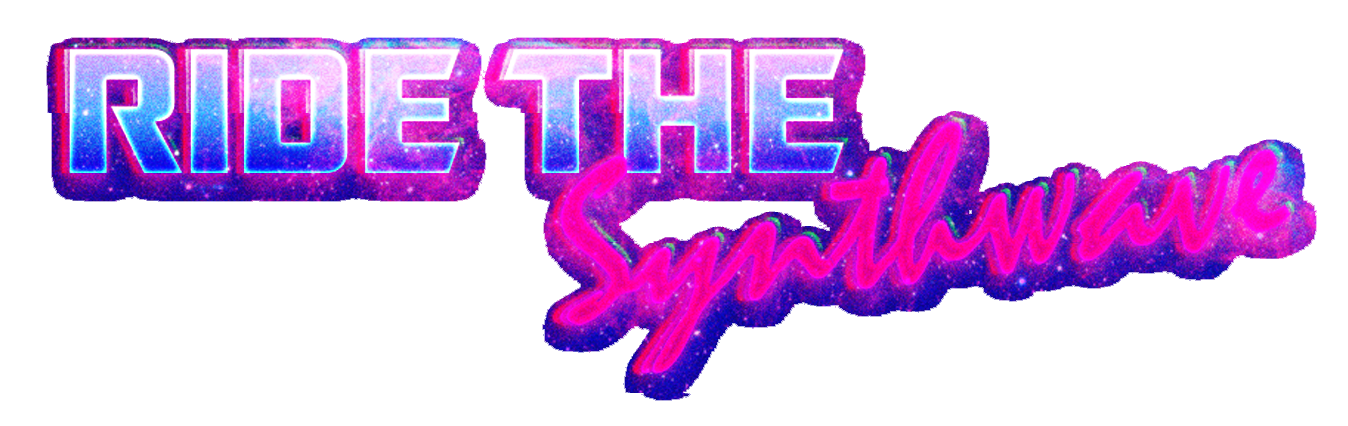The image showcases a highly stylized logo set against a completely white background. Centralized within the composition, the text "Ride the Synth Wave" is artfully designed with a blend of fonts and vibrant colors. The phrase "Ride the" is prominently displayed in the top left in a bold, capitalized font, sporting a dynamic gradient of white, blue, pink, and darker blue, evoking a galaxy-like theme with interspersed star-like elements. Just below it, in the bottom right, the term "Synth Wave" is elegantly scripted in cursive, rendered in a radiant neon pink, further enhanced by a blue-shadow effect that gives it a glowing, three-dimensional appearance. The overall aesthetic hints at the retro-futuristic "synthwave" genre, reminiscent of 80s and 90s digital culture, and suggests it could be part of an online graphic, possibly serving as a logo for a music-related project or a graphic design element for a website.